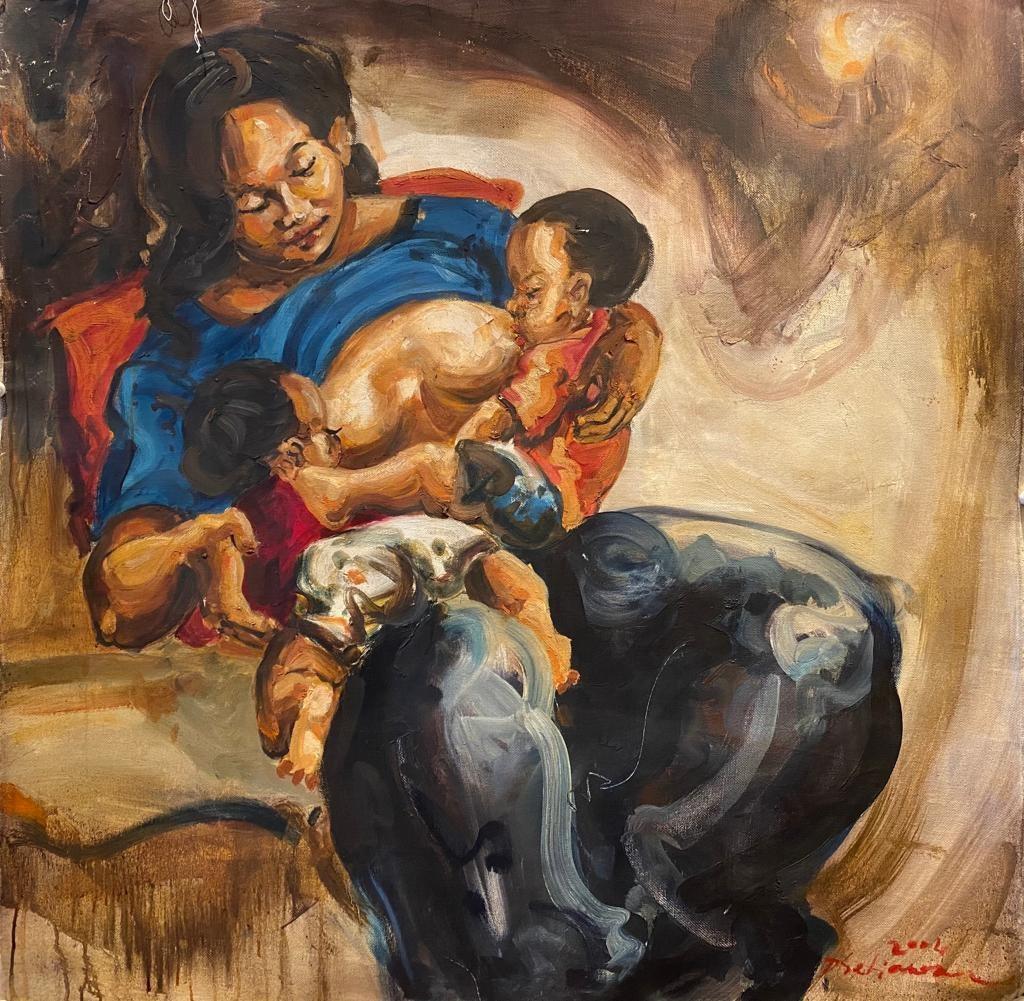In this vividly colorful painting, a mother with dark brown hair, possibly Latino, is depicted breastfeeding her twin babies, who are the same age. She is seated in a chair that has an orange-rose hue, wearing a blue t-shirt pulled up to expose her breasts, while she lovingly nurses her children. Her attire also includes dark pants. Each baby, dressed in a red top, is nestled on her lap: one with his legs stretched and kicking, the other with his legs straddling her. The mother's left hand clasps the leftward child, and her right hand holds the rightward child. The background consists of a mix of light tan, dark brown, and intermixed colors, creating a textured and dynamic backdrop. At the lower right-hand corner of the painting, there is a signature in red paint that is somewhat difficult to decipher, but the artist’s last name seemingly begins with the letter 'M'. In the top left, there's a white thread-like object hanging down, complementing the detailed portrayal of the scene.